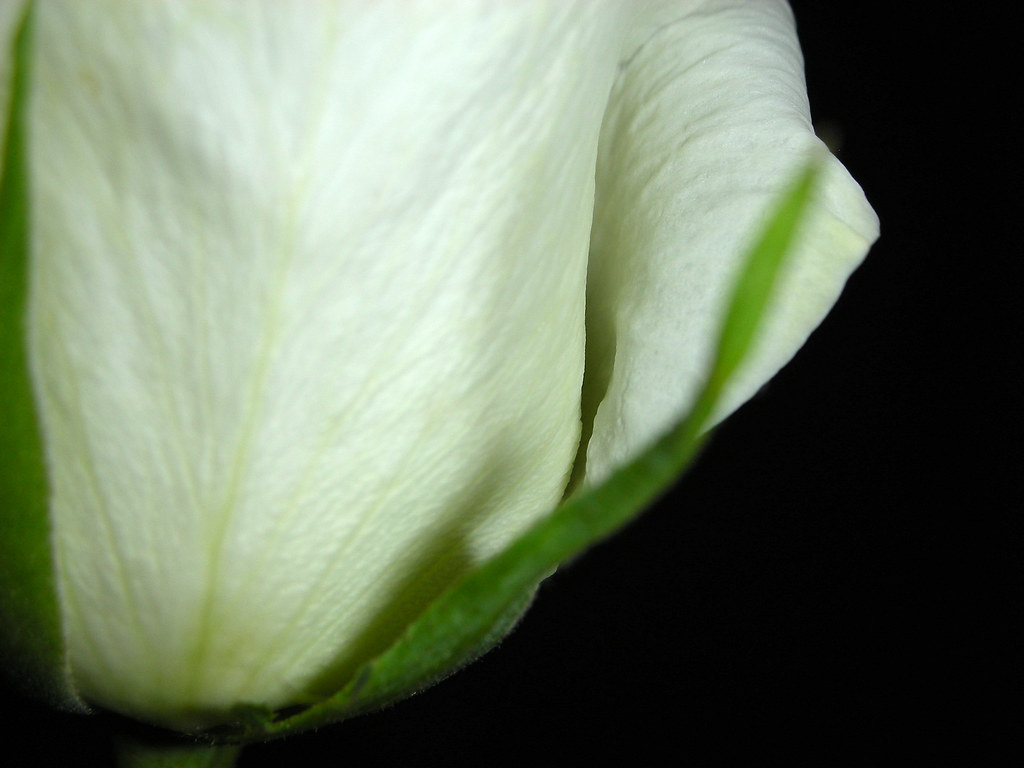This image is an extreme close-up photograph capturing a delicate leaf, likely from a piece of lettuce, set against a plain black background. The composition is minimalistic, highlighting the subtle beauty and intricate details of the greenery. The leaf exhibits a gradient of colors, starting with a very pale green at the center and transitioning to a richer, darker green at the edges. Central to the leaf, a thin, lime-colored line runs upward, fading as it moves to the center. The leaf appears to be folded over slightly on the right side, with hints of lime green accentuating its edges. Additional details include small grains and intricate lines within the leaf, as well as faint white or pale yellow spots near the base where smaller leaves branch out. The close-up view emphasizes the vibrant and crisp nature of the leaf, making the details and variations in color and texture stand out vividly against the stark backdrop.